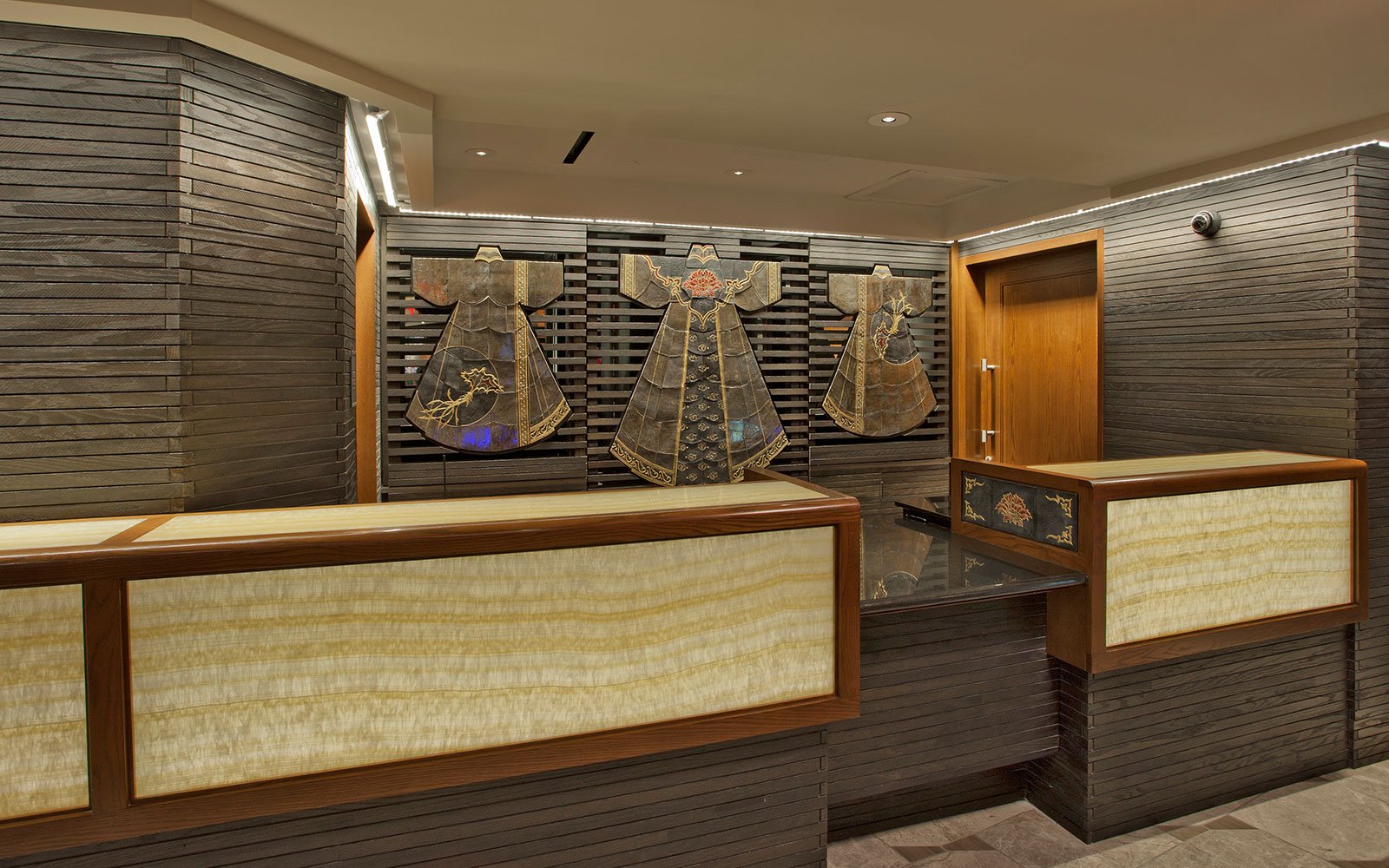The image depicts a sophisticated kiosk or reception desk, likely situated within a high-end hotel or resort. The counter features a smooth, dark wood frame with light wood panels and a matching light-colored countertop. The front of the desk is adorned with white and yellow marble-like lines, giving it a luxurious touch. Surrounding the desk, the walls are lined with very thin, long wooden slats that exude an elegant, contemporary feel.

Behind the desk, three ornately designed pieces of traditional Asian attire are prominently displayed against a backdrop of dark, ashy wood slats. The central garment is larger and more prominent, flanked by two slightly shorter pieces, all embellished with intricate gold designs and filigree ribbons. The outfits have an antique appearance, reminiscent of vintage kimonos, and may include bird illustrations, particularly on the outer two garments.

A small security camera is mounted on the wall to the right, near a light brown wooden door, adding a subtle element of surveillance to the space. The overall ambiance suggests a blend of modern luxury and traditional Asian art, making it an intriguing and unique setting.